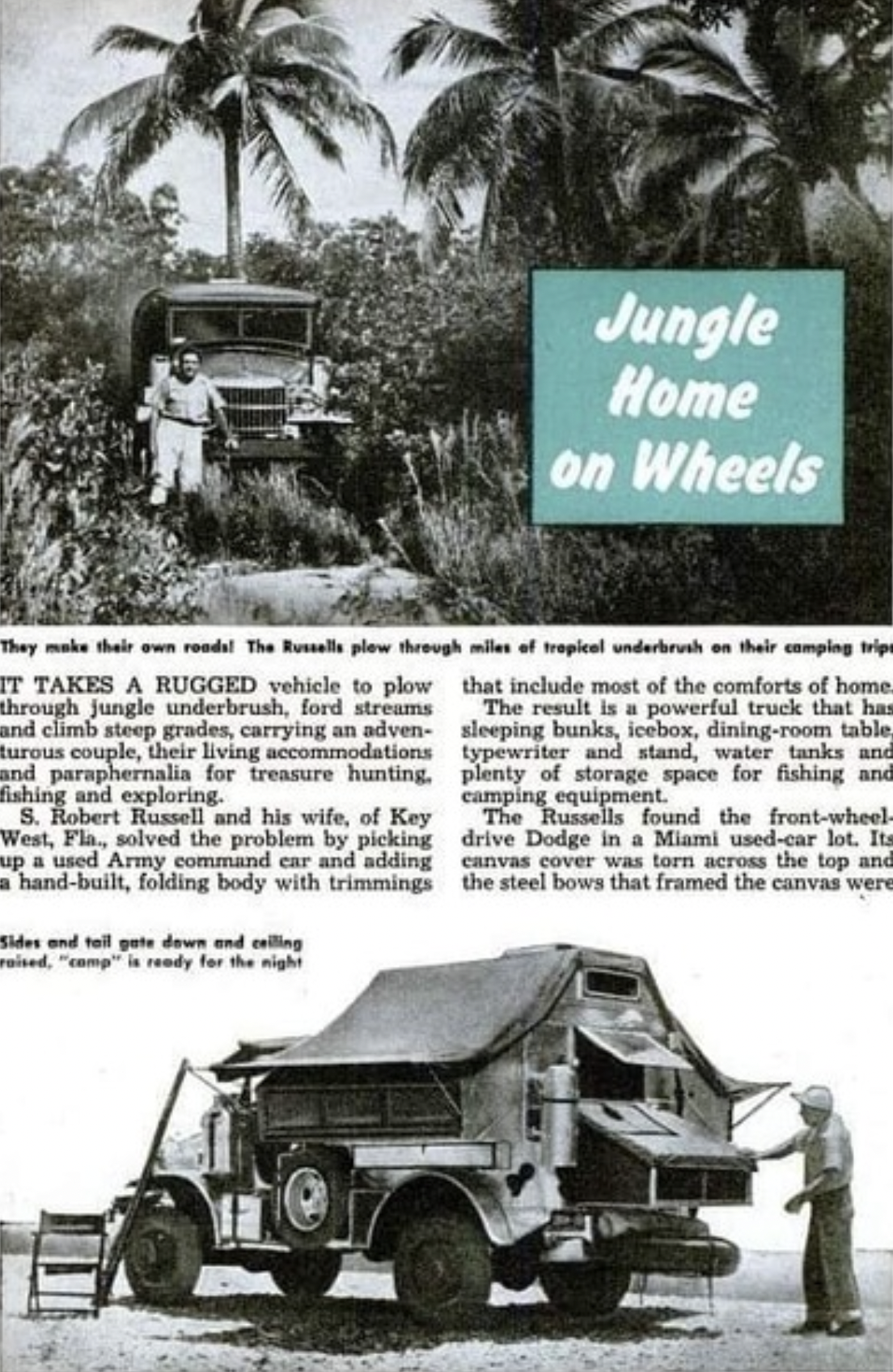This is an image of a page from an old magazine, evident from the black and white photography and the vintage attire of the people depicted. A prominent photograph at the top of the page shows a man standing next to a heavily customized vehicle in a jungle setting, with dense vegetation and palm trees in the background. The vehicle, either a truck or a car with a camper conversion, is designed for rugged terrain, supported by the text in a green (or muted blue) box that reads, "Jungle Home on Wheels." This box is the sole splash of color on the page. Below the main photo, smaller text begins an article detailing the adventures of a couple using this vehicle for treasure hunting, fishing, and exploring tropical underbrush. At the page's bottom, there's a close-up image of the back of the camper, revealing additional customizations like windows and possible metal structures, suggesting it's a makeshift home built for their journey.